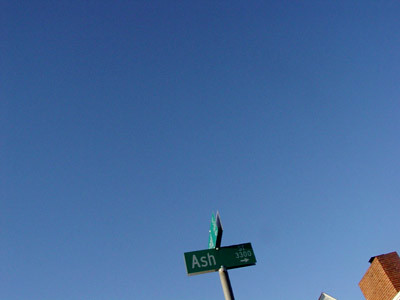The photograph captures a vivid, clear blue sky occupying 90% of the frame, devoid of any clouds. At the bottom, a street sign prominently displays the name "Ash" in bold, white letters on a green background, accompanied by the numbers "3300" and a small, right-pointing arrow. Above this, another green sign is visible, oriented perpendicularly, though its text is unreadable. In the photograph's top right corner, a small portion of a brick building is visible, with something black perched on its top edge. Nestled between the street sign and the building is a tiny sliver of a silver object.